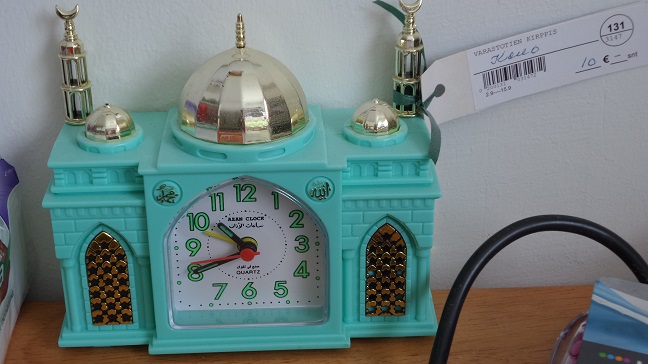This image features a uniquely designed clock resting on a wooden shelf with a plain white wall serving as the backdrop. The clock is styled to resemble a small church and is painted a striking turquoise blue. At the top of the clock is a small silver tower, flanked by two smaller silver towers on either side. Extending from the back of the clock are slender, silver rods that are open in the middle, ending in pointed, hook-like tips.

The clock face is white and prominently displays numbers 1 through 12 in green, which appear to possibly be luminescent. The time is indicated by black hour and minute hands, and there's a vibrant red second hand coupled with a yellow alarm hand. Each side of the clock is adorned with what appears to be a stained glass window design, crafted using gold and black, adding to the textured and ornate appearance.

Attached to one of the silver rods at the back is a tag. On the tag, a barcode is visible alongside a circle containing the number 131 and text that seems to spell "VARASTOTEN KARPRIS," although it is not completely legible. Additionally, there is a black tube situated to the right side of the clock, the purpose of which is unclear. A small, indistinguishable blue and white item appears near this tube. To the left of the clock, another white and blue object lies on the shelf, though its exact nature is also unclear.